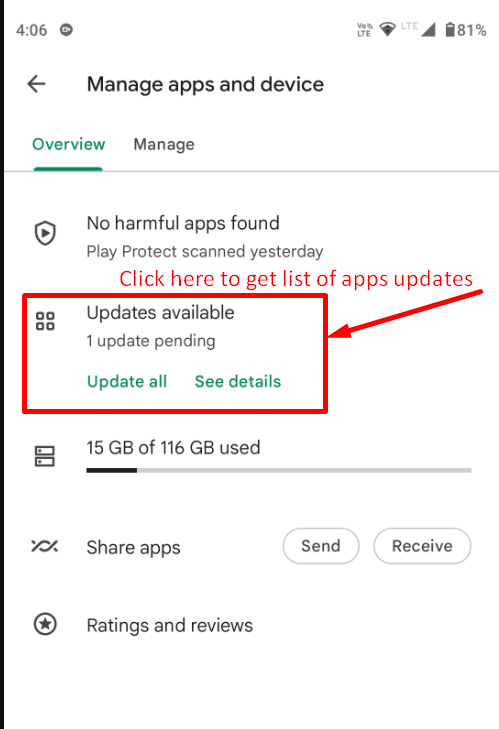This image seems to be a screenshot taken from a smartphone, displaying a portion of the interface related to managing apps and device settings. The layout includes several UI elements and icons.

- On the top left corner, there is a time display that reads "4:06," followed by a small, indistinct circle icon resembling a camera.
- The top right corner features connectivity indicators: the letters "LTE," a Wi-Fi icon showing approximately three-quarters signal strength, another instance of "LTE," a fully filled signal bar, and a battery icon displaying "81%" charge.
- Directly below these indicators, there is a navigation arrow pointing to the left, and centrally placed text that reads "Manage Apps & Devices."
- Just underneath "Manage Apps & Devices," the page is divided into two sections: "Overview" (which is underlined) and "Manage."
- Further down, there is a shield icon followed by the text "No Harmful Apps Found," with "Play Protect Scan Yesterday" indicated below it.
- Red text reads, "Click Here to Get Lists of Apps, Updates," accompanied by an arrow pointing to a box. 
- The section below states "Updates Available, One Update Pending, Update All," and possibly "CD Tips."
- A storage summary is provided, saying "15 GB of 116 GB used," illustrated with a progress bar.
- Options for "Go to Share Apps," and buttons labeled "Send" and "Receive" are included.
- Finally, "Ratings and Reviews" is listed at the bottom.

The left edge of the image is marked by a prominent black border, while the other sides remain unobstructed.